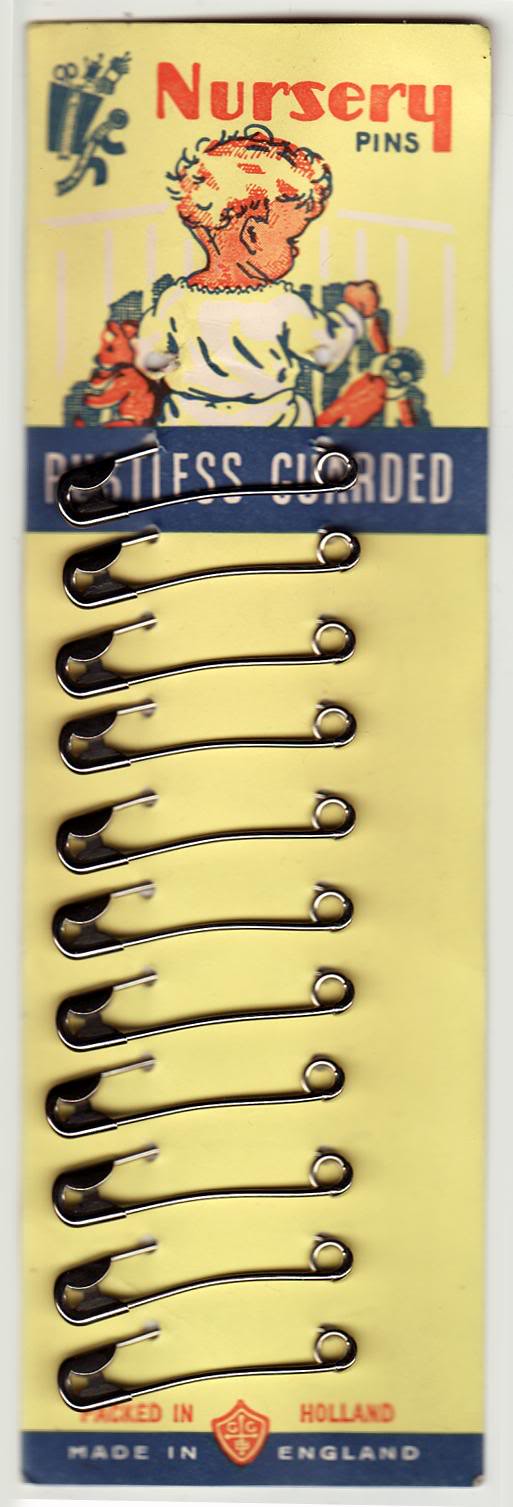This image depicts a vintage product tag for nursery pins, likely from the late 40s to mid-50s, emphasizing its old-fashioned design. The rectangular tag has a faded, light yellow background adorned with red, dark blue, and white details, giving it a nostalgic appeal. In the upper right-hand corner, there is clip-art style iconography featuring sewing tools like scissors and a measuring tape. Adjacent to this is red text reading "Nursery," and below that, blue text reading "Pins."

The header of the tag showcases a stamp-style illustration of a baby, depicted from behind with a head of hair, dressed in a white onesie or robe, and playing with a teddy bear. Below this illustration is a blue bar with white text that reads, "Restless Guarded." The lower part of the tag includes red text that states "Packed in Holland," flanked by a red shield symbol, and a blue bar at the very bottom with white text saying "Made in England."

Clipped to this cardboard tag are 11 silver-tone safety pins, aligned neatly. These nursery pins were historically used for securing cloth diapers, known as pampers, keeping them in place on babies. The overall aesthetic and detailed descriptions on the tag indicate its vintage nature and a specific era of manufacturing.